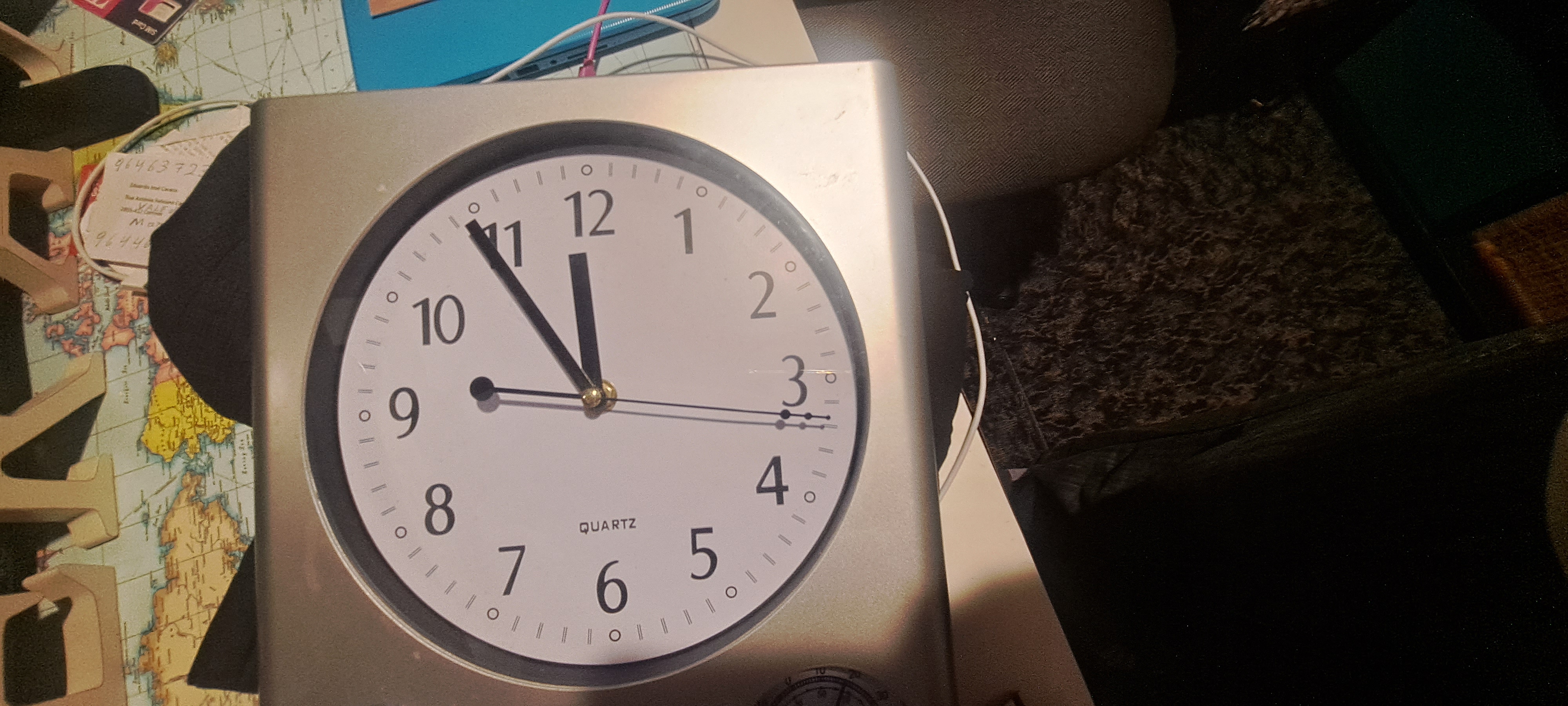The photograph appears to be taken inside a home, featuring a desk with a flat, detailed world map spread out on its surface. In the background, there are decorative wooden letters spelling out "EAT," made from a light-colored wood, reminiscent of common kitchen decor. Various objects are scattered across the desk, including what seems to be a blue shirt and possibly a computer.

Prominently displayed in the image is a clock with a light rose gold frame and a white face. The clock features distinctly black numbers ranging from 1 to 12, and exhibits a precise time of 12 o'clock, with the slender second hand positioned at 17 seconds. The face of the clock is illuminated by a strong artificial light source, creating a bright reflection on one spot.

Towards one side of the image, there is a square object adorned with a dark floral pattern. The lighting in this section is dimmer, making it difficult to discern the finer details of this item. Additionally, several wires are visible beneath the desk, adding to the sense of a lived-in, functional space.